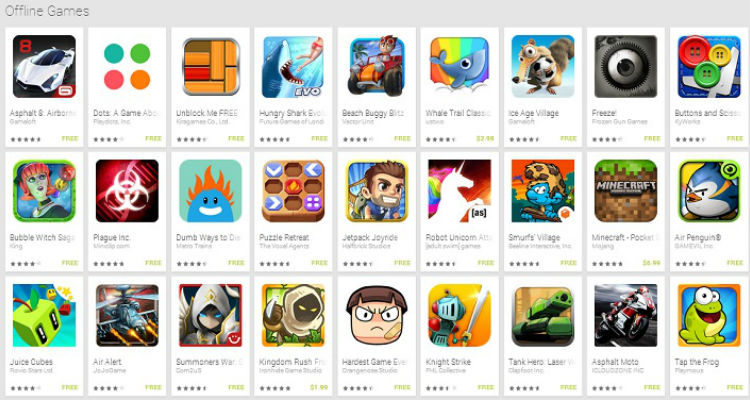This image is a screenshot from a mobile play store's game section, likely from an Android or similar platform. The interface features a gray navigation bar at the top. In the upper left corner, "Offline Games" is written in gray font.

Below the navigation bar, there are three horizontal rows, each displaying nine games. Starting from the upper left corner of the first row, the games listed are:

1. Asphalt 8: Airborne
2. Dots: A Game
3. Unblock Me Free
4. Hungry Shark Evolution
5. Beach Buggy Blitz
6. Whale Tail Classics
7. Ice Age Village
8. Freeze
9. Buttons and Scissors

Following on the second row from the left:

1. Bubble Witch Saga
2. Plague Inc.
3. Dumb Ways to Die
4. Puzzle Retreat
5. Jetpack Joyride
6. Robot Unicorn Attack
7. Smurf Village
8. Minecraft Pocket Edition
9. Air Penguin

And on the third row from the left:

1. Juice Cubes
2. Air Alert

The games are displayed with their icons and titles, providing a comprehensive view of various offline games available for download.